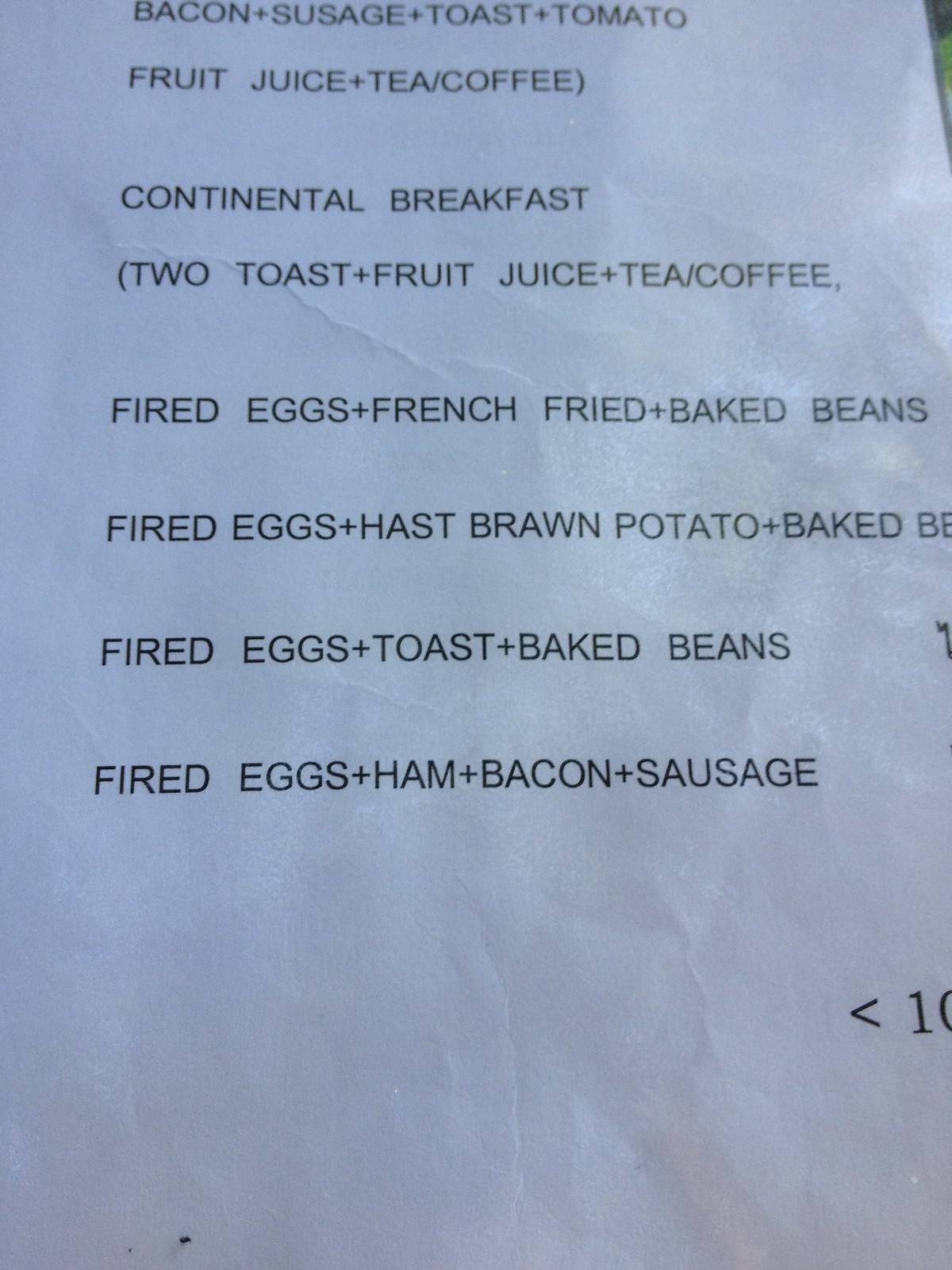The image showcases a hand-written menu listing various breakfast foods in black ink on a white piece of paper with a noticeable blue tint. It is unclear whether the blue tint is due to ambient lighting or if the paper itself is blue. The listed breakfast items begin at the top of the page, which is partially cut off, suggesting there may be more foods not fully visible in the image. The listed foods include "bacon sausage," "bacon + sausage + toast + tomato," and "fruit juice + tea/coffee." The items continue with "continental breakfast," "fired eggs," "French fried," "baked beans," and "fired eggs, toast, and baked beans," where "fired" appears to be a misspelling of "fried." At the lower part of the right edge, there is a ">" symbol followed by the number "10." The page also displays crinkle marks, especially in the unscribed areas, adding to its texture.